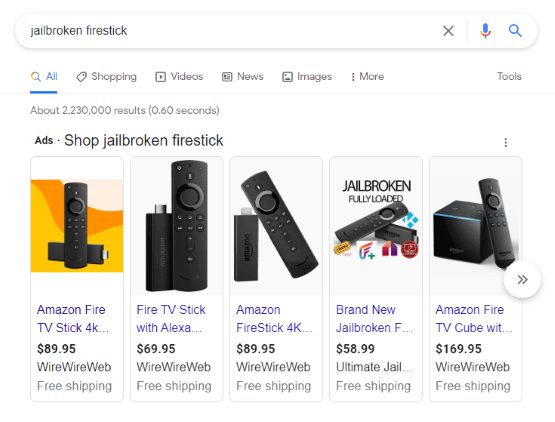This screenshot, taken from a Google web browser on a computer, offers a cropped view that omits some broader context, yet distinctly showcases a Google search tab. The search term "jailbroken fire stick" has been entered, and the results focus on the top shopping options available. Displayed prominently are five images of Amazon Fire Sticks, a product designed for streaming TV. These results, sourced from the shopping site WireWireWeb, list various models of the jailbroken Fire Stick with prices that range from $69.95 to $169.95. The distinct color scheme of the browser and the layout of the shopping results underscore the nature of the search and the online marketplace context.